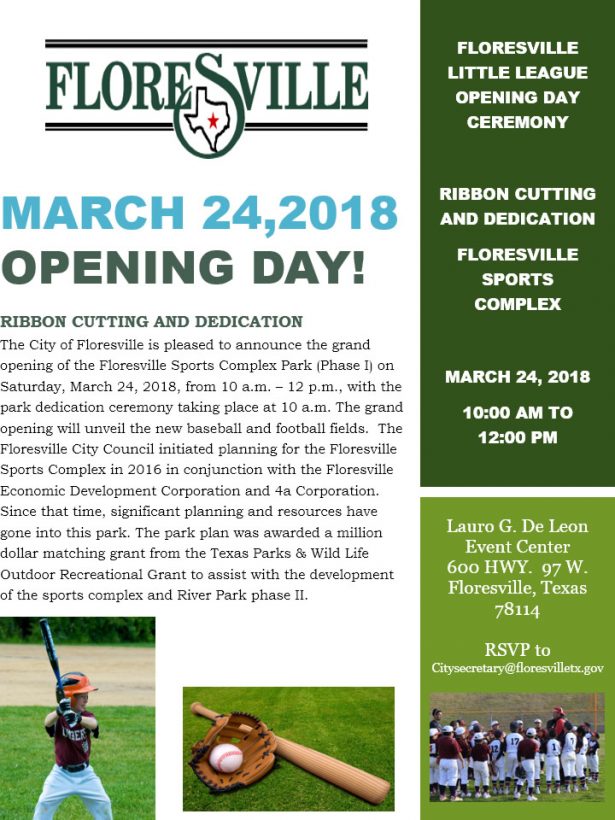The image is an advertisement for the Floresville Little League Opening Day Ceremony, scheduled for March 24th, 2018, from 10 a.m. to 12 p.m. at the Floresville Sports Complex. The event includes a ribbon-cutting and dedication ceremony. At the top, the advertisement features a logo with the text "Floresville." It prominently highlights the details of the event in a green-bordered section, including the venue’s address: Laurel G. DeLeon Event Center, 600 Highway 97 West, Floresville, Texas 78114. Attendees are invited to RSVP to the City Secretary at FloresvilleTX.gov. The image includes three photos: one of a young boy holding a bat, preparing to play; another of a bat, ball, and glove on the grass; and a team photo of Little Leaguers. The advertisement also mentions that the ceremony will unveil the new baseball and football fields, developed with a significant grant from the Texas Parks and Wildlife Outdoor Recreational Grant as part of the Floresville Sports Complex Park Phase 1, planned in conjunction with the Floresville Economic Development Corporation and 4A Corporation.